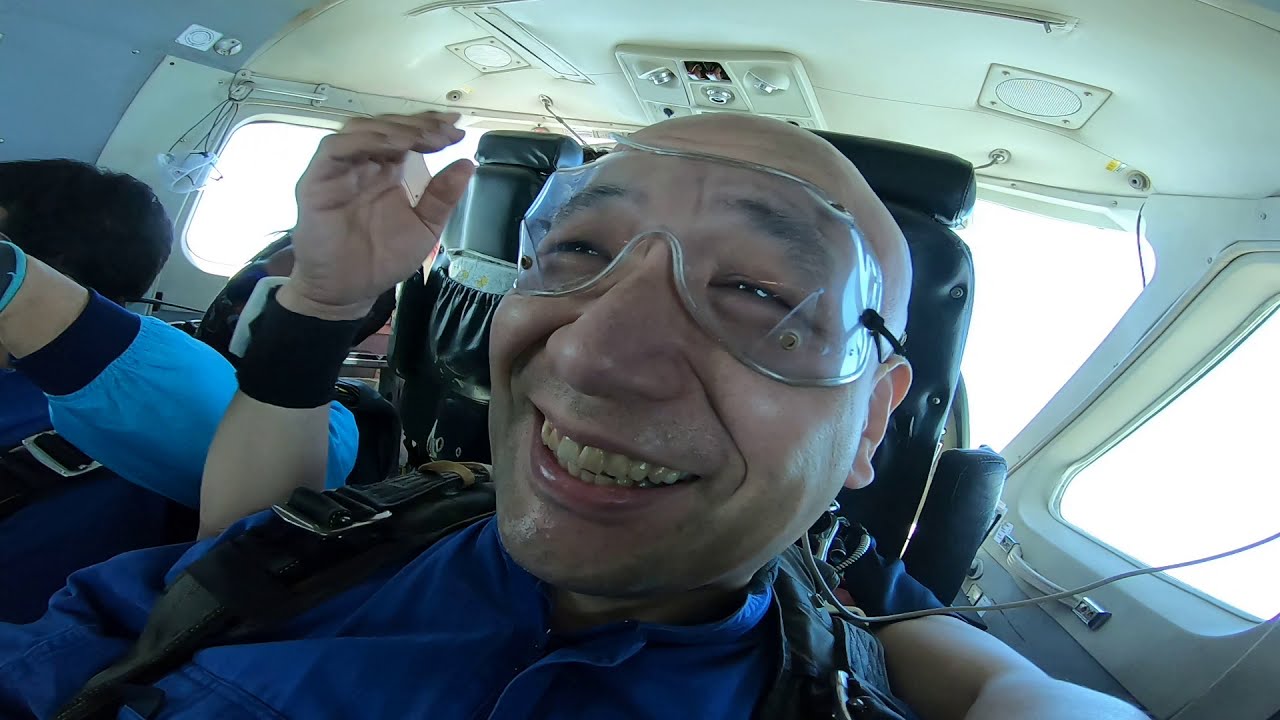This image is a close-up selfie taken by a smiling, bald man inside a tightly enclosed vehicle, likely an aircraft. He is wearing transparent glasses and a blue shirt with black straps around his shoulders, suggesting he may be equipped with a parachute. To his side sits another individual in a blue shirt whose face is obscured by a hand. Behind the main subject, other people can be seen, including one with a raised hand. The interior of the vehicle is entirely white, with various instruments attached to the ceiling. The windows appear bright white, obscuring any view of the exterior.